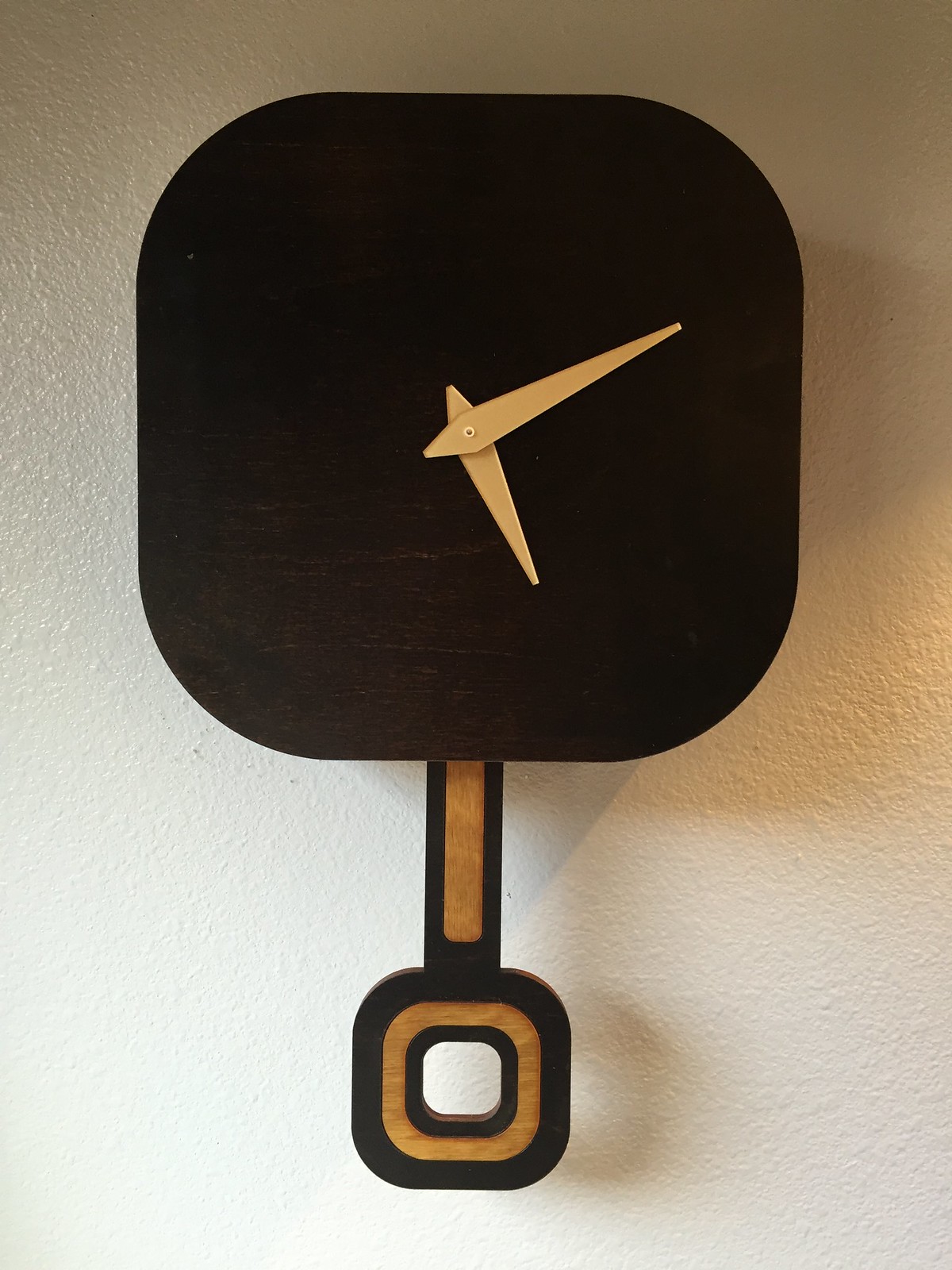A minimalist clock with a sleek, modern design is showcased in this image. The clock features a squircle-shaped face—a square with elegantly rounded edges—enhancing its minimalist appearance. The dial is starkly simple with no numbers or second hand, only displaying the minute and hour hands for a clean and uncluttered look. The clock is mounted on the wall by a minimalistic vertical bar that discreetly anchors the clock beneath its face, emphasizing the aesthetic of simplicity and functionality.